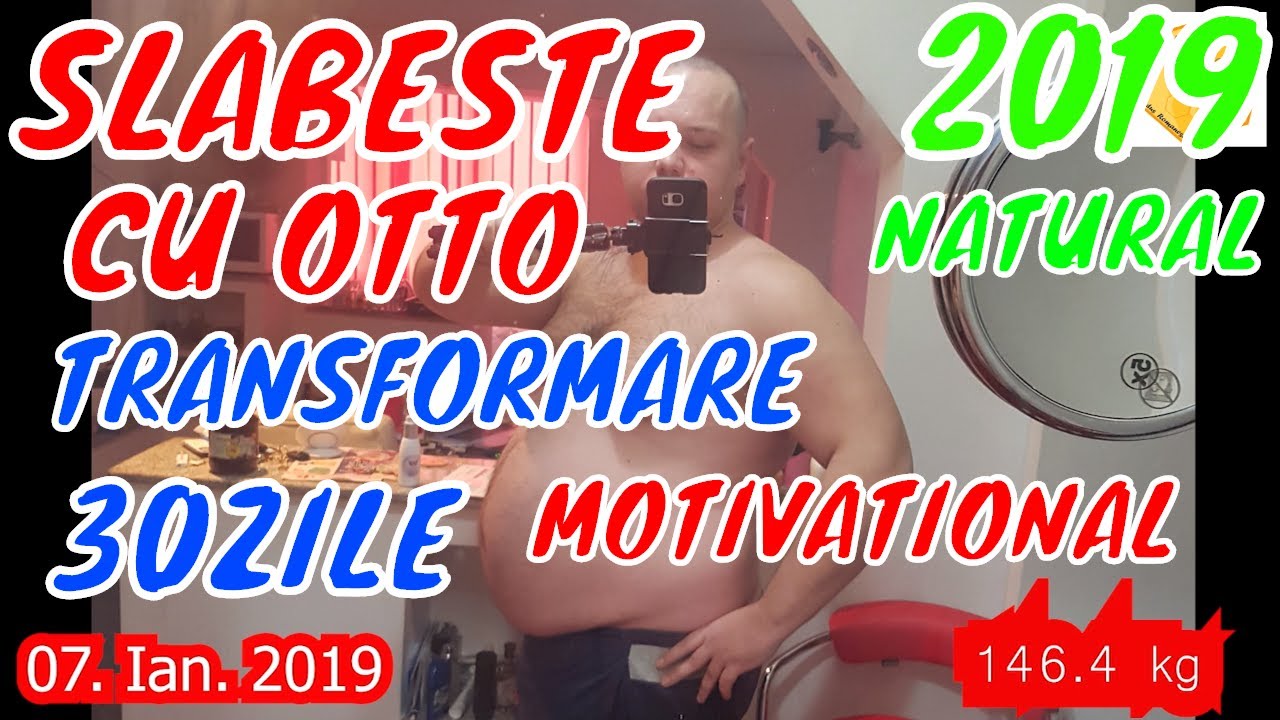In the center of the image, a half-legged, shirtless man stands sideways with his belly facing left, prepared to take a selfie. His left hand rests on his hip, and he holds a black cell phone equipped with a selfie stick in his right hand. He looks at himself intently. The room behind him features a window with a pink blind, in front of which sits a white desk cluttered with various items, including a brown container and a white bottle near the edge. Text overlays in multiple languages and colors are present: "Slabesti Cu Ato" in red, "Transformer 30 Sili" in blue, and "2019 Laptro" in bright green at the top right. The bottom right corner includes the motivational text "146.4 kg" in red, while the bottom left corner shows the date "07.01.2019" in white font highlighted in red.